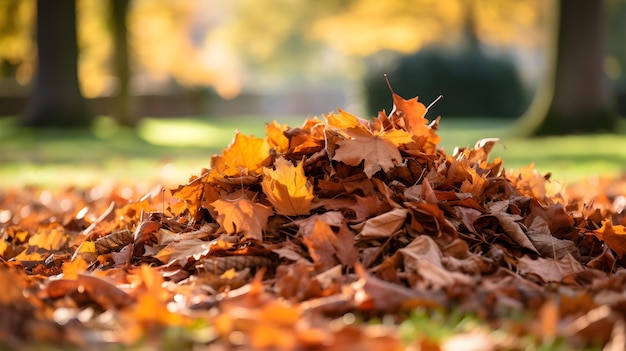The image depicts a scene on a sunny autumn day, capturing an open area with a ground covered in green grass and patches of dried leaves. In the center, there's a not very large, but well-defined pile of leaves, mostly golden brown, suggesting they have fallen and aged over time. Amid this pile, a few pine cones are visible towards the bottom left. The surrounding ground has more scattered leaves, adding to the seasonal ambiance. The backdrop features a blurred view of trees, with leaves in shades of yellow, orange, and brown, echoing the colors of the central pile. The sunlight, seemingly coming from behind the scene, enhances the rich autumnal hues, indicating that this photo was likely taken in the late afternoon during the autumn months.